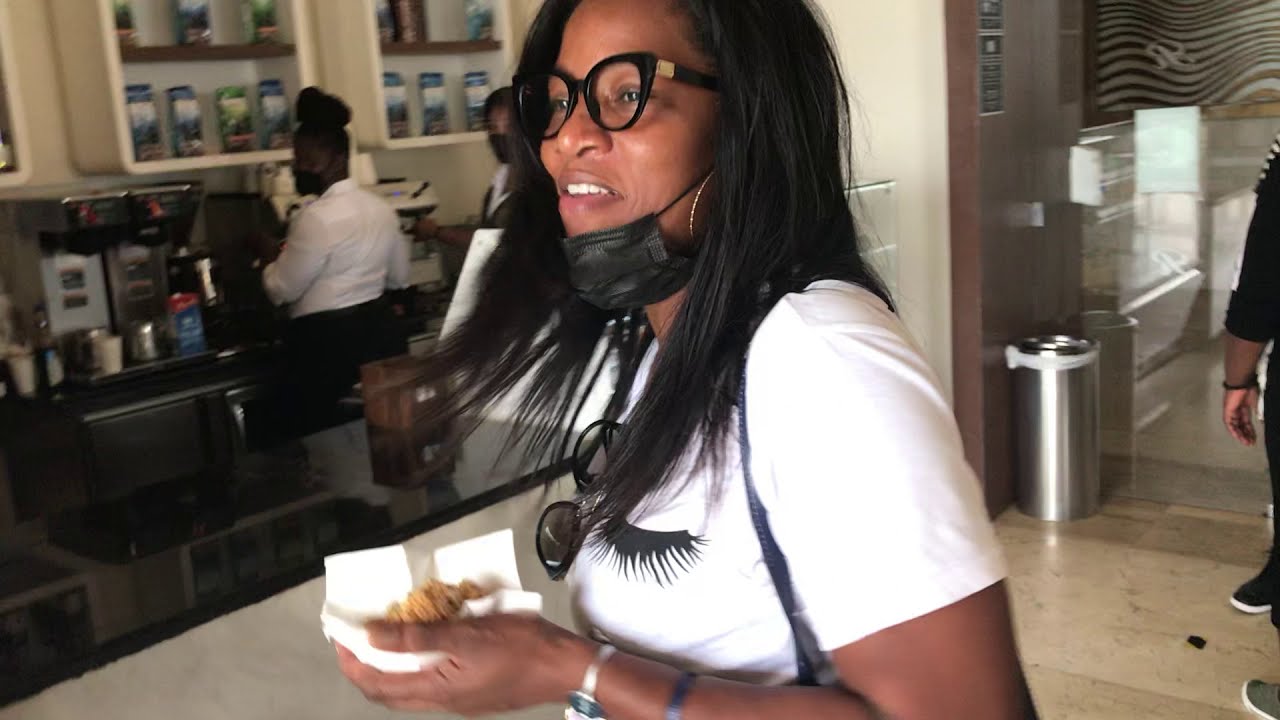In this image, we see an African-American woman centrally positioned inside a chic, modern cafe. She has long, straight black hair cascading forward, wears large, thick-framed sunglasses sitting on top of her head, gold hoop earrings, and a white short-sleeved t-shirt with a design featuring black eyelashes. She holds food in her hand wrapped in white paper, possibly cookies, and her black face mask is lowered to her chin. The cafe is spacious, with a light beige, marbled floor and brown and white interiors. A sleek, black marble countertop with a white base stands in the background, behind which various coffee machines are placed. Two African-American women employees in white uniforms with black pants and face masks can be seen behind the counter. The setting includes a shiny silver cylindrical trash can against a brown wall, a microwave, a black table, and shelves filled with an assortment of coffee packages, contributing to the cafe's well-equipped and stylish ambiance.